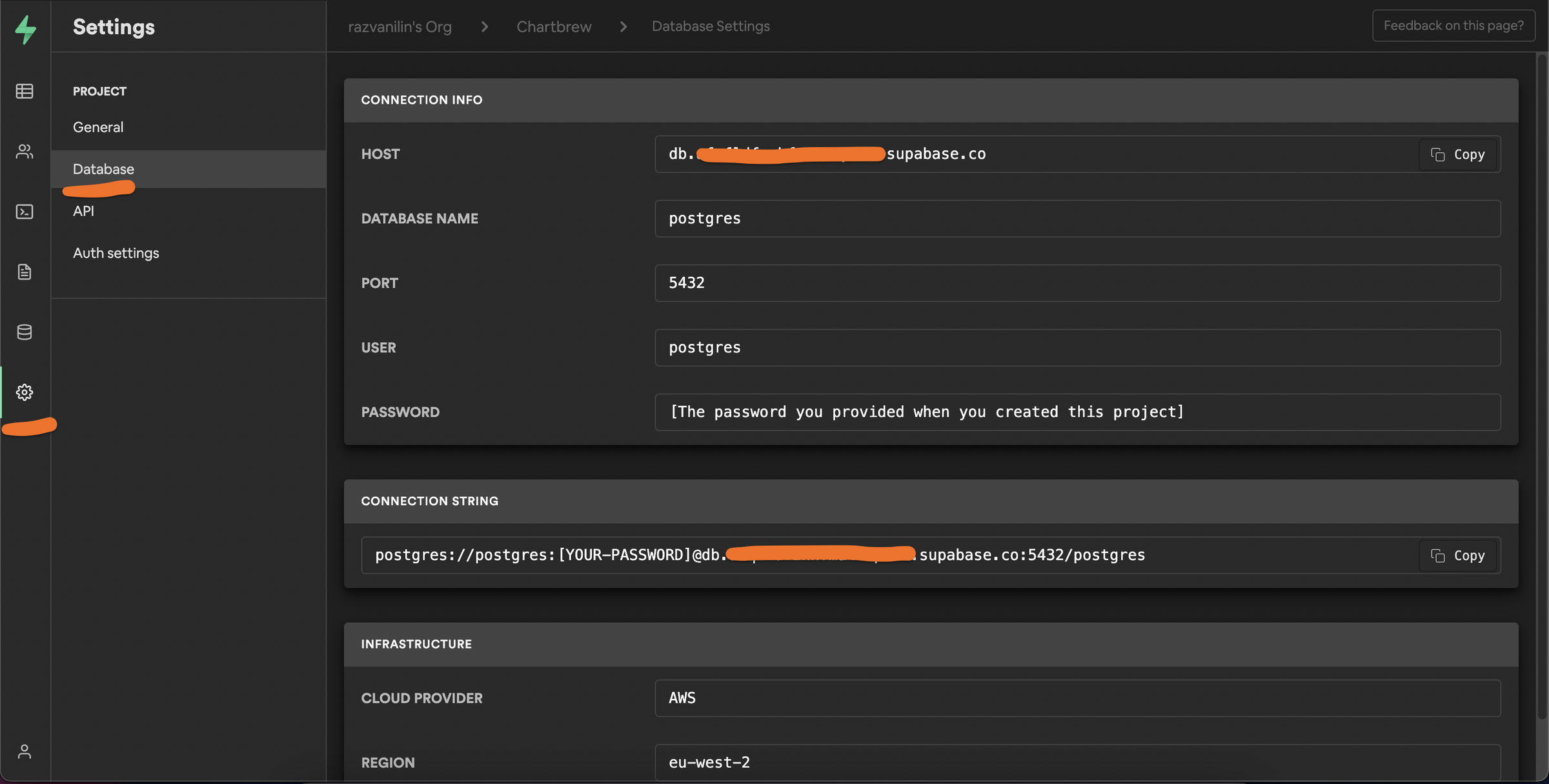The image displays a dark-themed settings page for an application. At the top left, in white text, the word "Settings" is prominently displayed. Below this heading, there is a vertical list of tabs labeled "Project," "General," "Database," "API," and "Auth Settings," with the "Database" tab highlighted in orange.

On the left side of the page, there are various icons: a green lightning bolt symbol at the top, an image icon, icons depicting two people, and a gear icon that is also underlined in orange.

At the top right of the page, the URL "razvinylins.org" is accompanied by arrows pointing to "ChartBrew" and then to "Database Settings." Below this navigation string, there is a chart titled "Connection Info." The first field in this chart is labeled "Host," next to which is a field partially obscured by an orange line, revealing text that reads "superbased.co." Subsequent fields are labeled "Database Name," "Port," "User," and "Password," each with corresponding input fields.

Further down, another section titled "Connection String" contains a text field with some input. The final section, labeled "Infrastructure," includes fields for "Cloud Provider" and "Region."